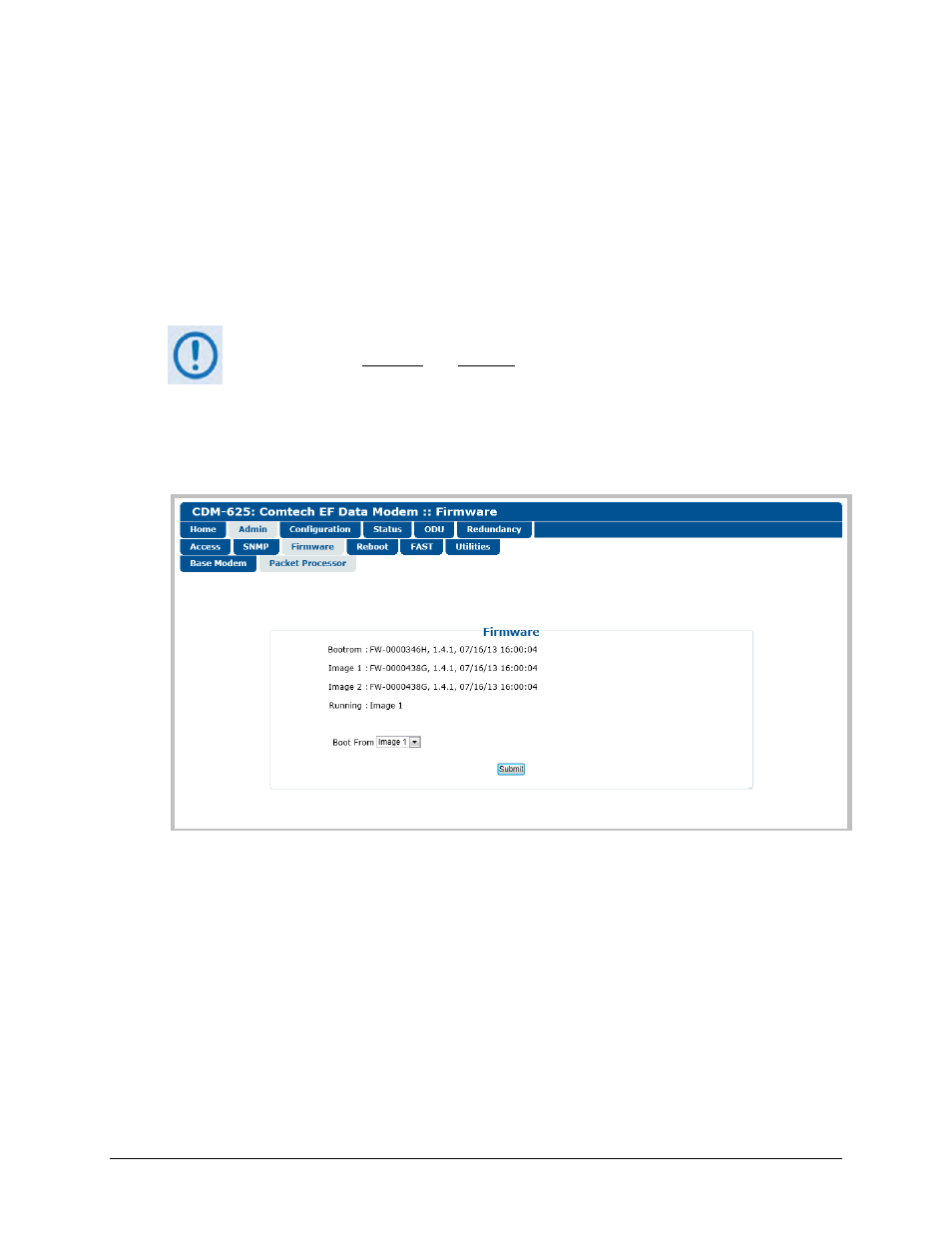Detailed Caption:

The image is a screenshot of the backend interface for a device management system, specifically for the CDM-625 ComTek EF Data Modem Firmware. At the top left corner, there is a grey square featuring a blue circular icon with an exclamation point, signifying an alert or important information. To the right of this icon are two small horizontal black bars, likely representing additional menu options or minimization controls.

Dominating the center of the screenshot is a grey box with a prominent blue header that reads "CDM-625 ComTek EF Data Modem Firmware." Below this header, several blue-tabbed menu options are visible, including "Home," "Admin," "Configuration," and "Status," which appear to facilitate navigation and management of the modem's firmware settings and status monitoring. The interface is organized and seems designed to provide administrators easy access to various functionalities of the device.